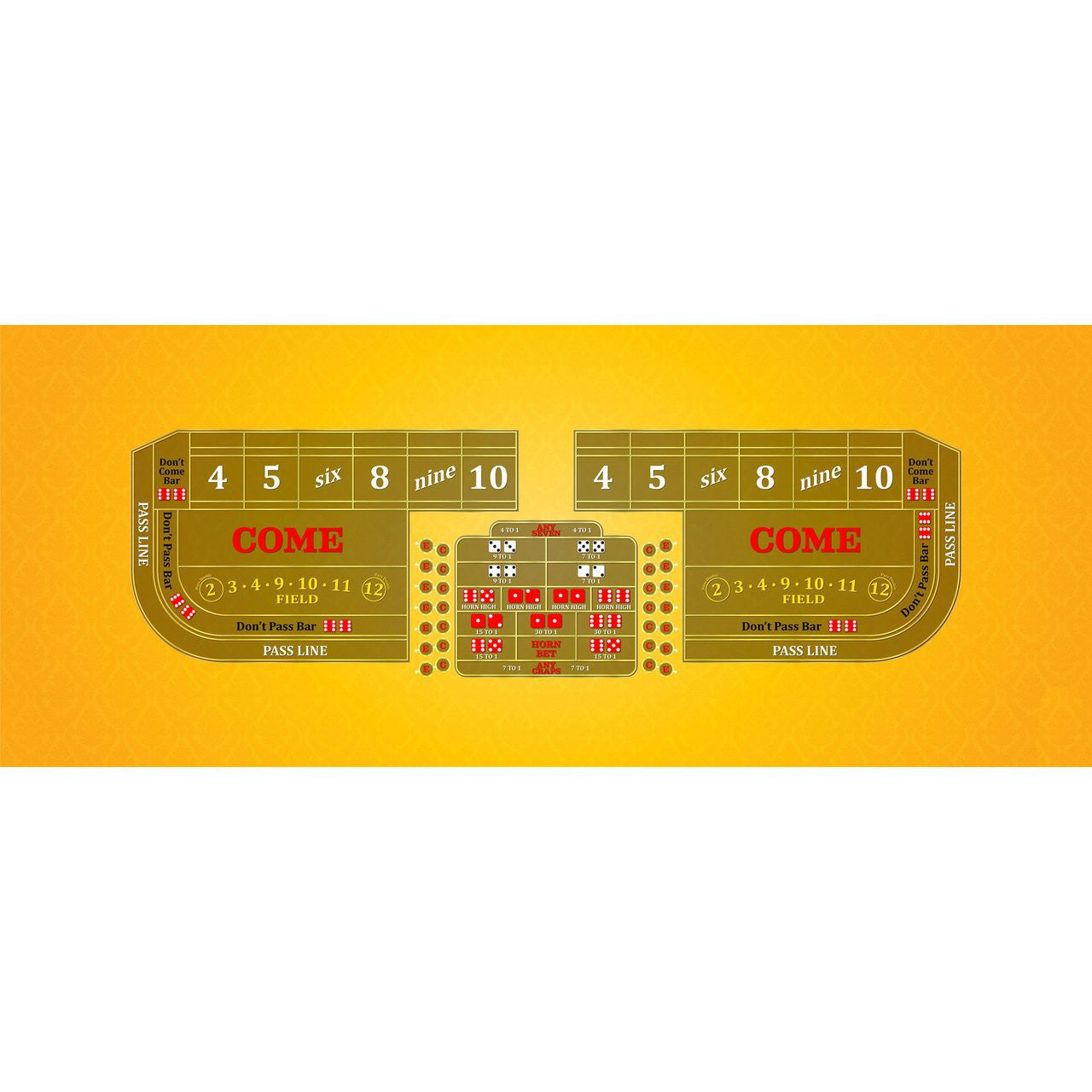The image depicts a rectangular game board, resembling a casino table game, set against a gradient background. The background transitions from a bright whitish-orange center to darker orange edges. The game board, divided into three sections, features curved corners on the bottom left and right. The board is filled with text and numbers including "Pass Line," "Don't Come Bar," "Don't Pass Bar," and numbers ranging from 2 to 10. These elements are mirrored on both sides of the board. The color palette includes gold, brownish yellow, red, white, and black. Centrally placed dice icons add to the casino-like appearance. The text and numbers on the board, printed in white and red, make it clear that this is a detailed representation of a casino table game, likely a form of craps.